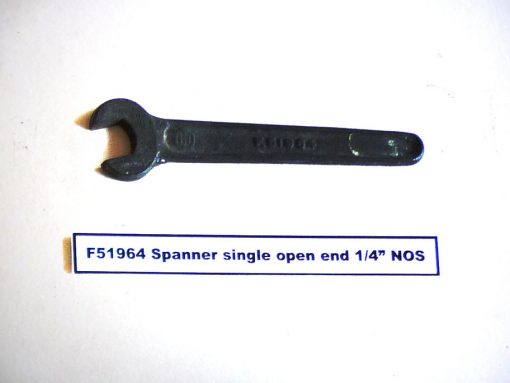The image prominently features an old-fashioned black spanner, positioned centrally on a bright white background, which could be a table or sheet illuminated by strong light. The spanner, made of metal, likely steel or iron given its black color and surface scratches, has an open end on the left and a long handle extending to a curved end on the right. Despite some raised letters and a logo in the middle of the handle, they are too small to identify clearly. Below the spanner, there is a white label bordered in navy blue with navy blue text that reads: "F51964 Spanner Single Open End 1/4 Inch NOS," with the letters "NOS" in all capitals. The spanner and label are centrally aligned, and both cast a subtle shadow to the left, adding depth to the image. The overall color scheme includes shades of white, black, and blue.